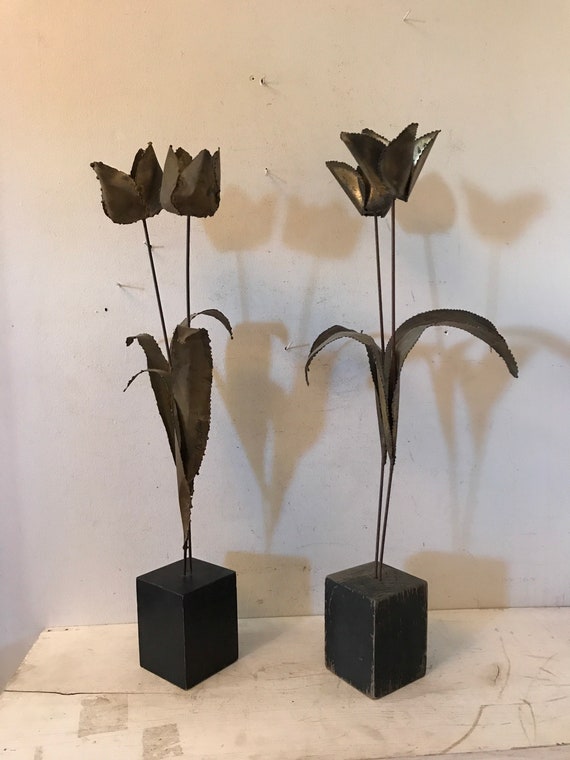The image depicts an indoor scene featuring a weathered wooden table or bench set against a white beige cream wall with hints of blue in its texture. On the table, two black decorative structures are prominently displayed. Each structure consists of a black cube base from which long, thin metallic pins protrude, adorned with fabric or metal leaves that extend outward. The top of each pin features metallic flowers, with two flowers on each structure displaying varying degrees of bloom. The left structure has partially opened flowers, whereas the right one showcases flowers in fuller bloom. The structures, resembling the silhouette of a rose, cast distinct shadows on the wall behind them, adding depth to the composition. The table’s surface appears scratched, cracked, and somewhat dirty, emphasizing a rustic or worn aesthetic.